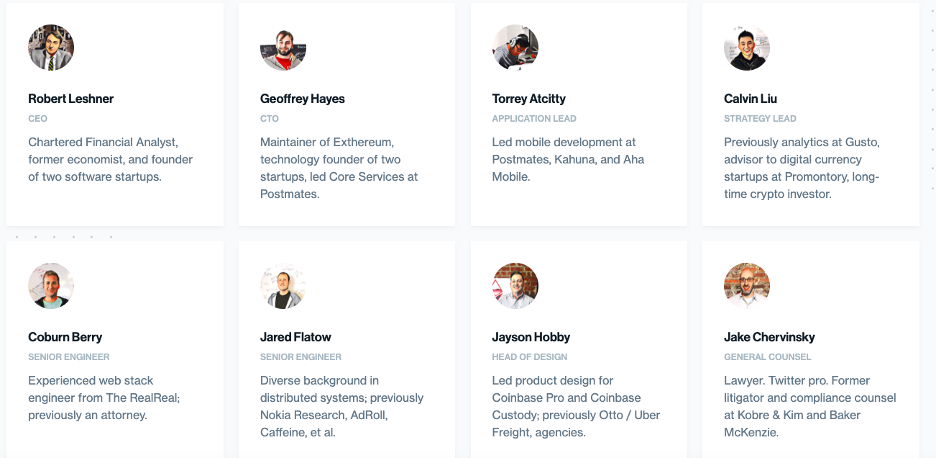The image depicts a grid of white rectangles set against a light gray background, each containing a circular portrait and corresponding names of different individuals. The first rectangle features a man in a suit and tie, identified as Robert Leshner, with small, unreadable text beneath his name. The second rectangle shows a man with a beard and mustache, dressed in a red t-shirt layered with another shirt, named Jeffrey Hayes. Next is a faintly visible portrait labeled Tory Atoltty. Following this, the square shows a man in a black shirt named Calvin Luu.

On the subsequent row, the left rectangle contains a man labeled Corburn Berry. To his right, the next rectangle shows Jared Flatlow, whose portrait includes his shoulders. Further right is Jason Hobby, pictured in front of a brick wall. The final rectangle features a bearded man named Jake Chervinsky.